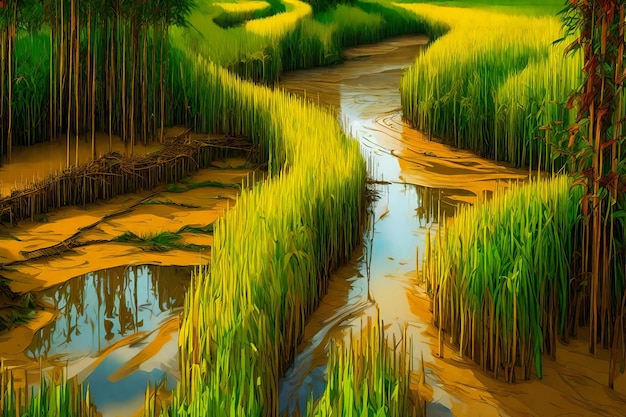This is a detailed, computer-generated graphic in landscape mode depicting a small, meandering river running through a vibrant bamboo forest. The water, which twists in an S-shaped path before branching into a Y towards the forefront, is a light muddy brown, with visible swirls of mud and a slight oily film on its surface. Reflections of tall, thin trees and thick, winding rows of yellow-green grasses add to the complex visual texture of the scene. On either side of the river, the bamboo stands tall, showcasing bare brown stems at the base with lush green leaves at the top. These plants grow closely together, creating a dense and immersive forest scene. The overall palette of the image includes the light muddy brown of the river, the vibrant yellow-green of the grasses, and the rich greens and browns of the bamboo forest under a sunny sky.